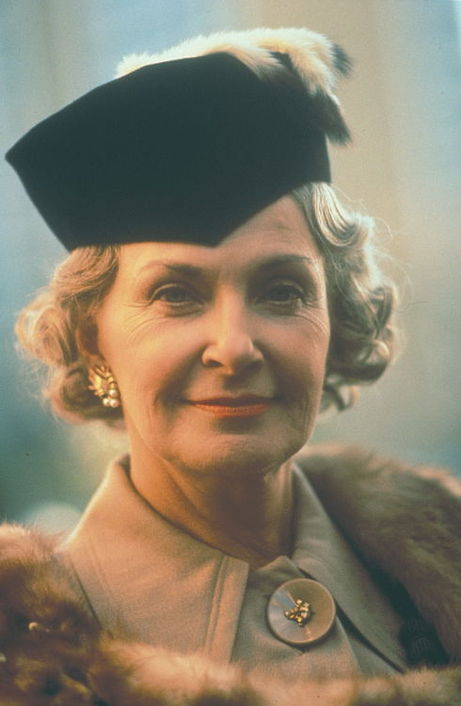This is a detailed photo of Joan Woodward, showcasing her in an elegant, period-style outfit that exudes upper-class European fashion. She dons a black hat adorned with white animal fur that has striking black tips. Joan's hair is styled short and fluffy, finished in an older, historical manner. She wears a luxurious brown and gray fur coat, which adds to her sophisticated appearance. Her makeup includes vivid red lipstick, complementing her slightly smiling expression as she gazes straight ahead. Gold earrings with pearls enhance her poised aesthetic, and a pendant can be seen adorning her attire. The background of the photo remains blurred and obscured, with vague hues of blue and orange, focusing all attention on Joan herself. The photograph has a portrait orientation, capturing Joan’s face and shoulders in close-up detail.